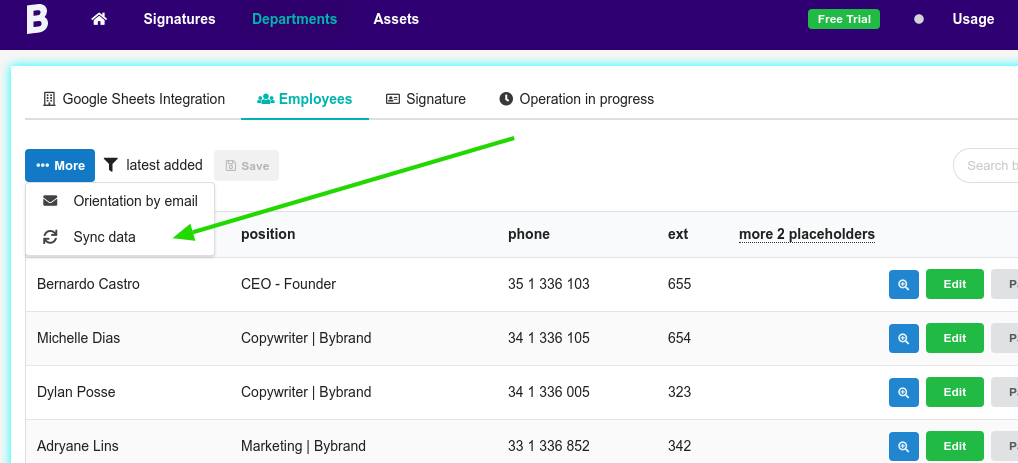This is a detailed screenshot of a management interface titled "Signatures," featuring a purple background. In the upper-left corner of the header menu, there is an italicized "B." The header menu includes options such as a home icon, "Signatures," "Departments" (highlighted in blue), "Assets," a green "Free Trial" button on the far right, and a "Usage" option. 

Below the header, the screen displays information on "Google Sheets Integration" and mentions that an "Employee Signature Operation" is in progress. The "Employees" section is highlighted. A long green arrow extends from "Operational Progress" down to an area labeled "Sync Data." 

Further down, a blue button labeled "More" leads to additional options including "Latest Added," "Orientation by Email," and "Sync Data," which appear as drop-down options. 

Headers on the interface include "Sync Data," "Position," "Phone Extension," and "More to Placeholders." Below these headers, there are entries for various employees, such as:
- Bernard Castro, CEO Founder
- Michelle Diaz, Copywriter
- Dylan Pose, also described similarly to Michelle Diaz
- Adrian Lins, Marketing By Brand

Each entry includes their respective phone numbers and three-digit extensions. Next to the names are blue, square search buttons and green edit buttons. Additionally, there is another button that starts with the letter "P."